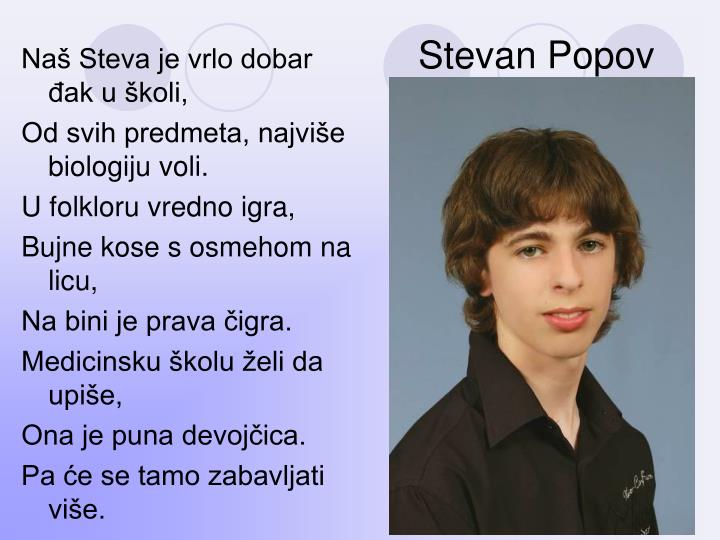The image features a teenager named Stephen Popoff, with short wavy hair and a headband, staring straight ahead. He is dressed in a black shirt with white text on the left side of his chest. The background is light blue and contains multiple elements: on the left side, there is a paragraph in a foreign language starting with "N.A. Lestiver Gerello Dabadauskaly" and ending with "Pachacetamo Sabavijati Vise." The image also includes additional sections of repeated text and a series of five circles at the top, shifting between the left and right sides.